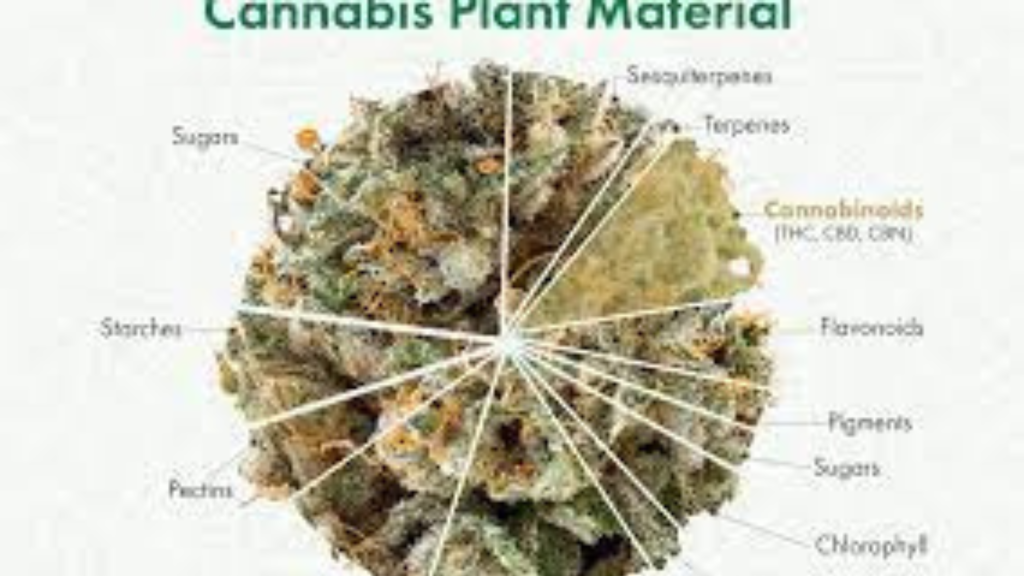The digital poster displays a low-quality image with unclear text and a blurry picture, possibly representing the components of a cannabis plant. At the top of the poster, "Cannabis Plant Material" is prominently written in large green letters. Below the title, there is a circular close-up photograph of a cannabis bud featuring a mix of green, yellow, and brown colors, and accented with white lines. Surrounding the circular image are various labels with arrows pointing towards specific parts of the bud, identifying components such as sugars, starches, chlorophyll, terpenes, cannabinoids, flavonoids, pigments, and other chemical elements. The background of the image is light gray, creating a contrast that highlights the text and diagram.